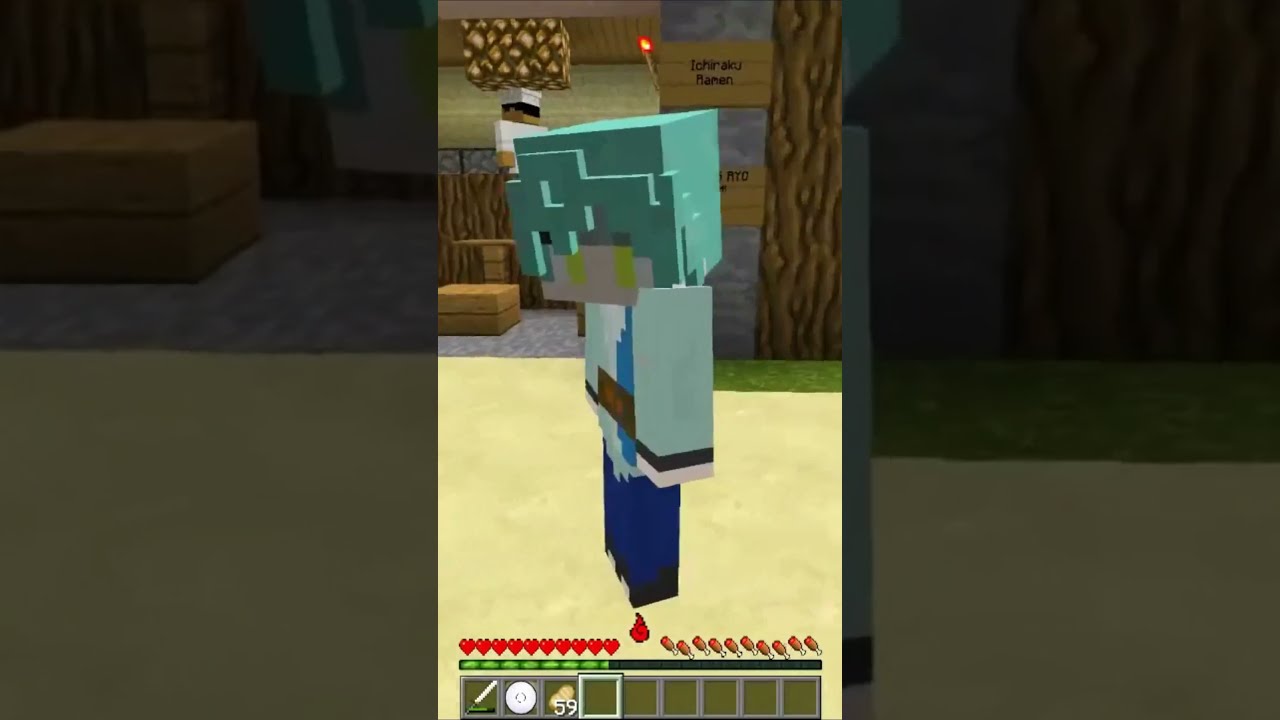This image is a screenshot from a video game, likely resembling Minecraft. The screen is divided into three vertical segments, where the central segment is more prominent with a yellow backdrop. In this segment, a character with a large, teal-blue 2D head and a blue rectangular body stands in the middle. The character’s head is angled slightly and the body is composed of blue, brown, and white blocks. At the bottom of this central segment, there is a row of heart icons and other items typically used in gameplay. 

The left and right segments of the screen show darker versions of the same scene, possibly indicating peripheral vision or split-screen elements. Behind the central character, the background features a beige ground with brownish elements that may represent a sandy, forest-like terrain. Off to the right, there's a tree, while to the left, the upper part of another character dressed in white is visible. 

Also in the background, a small panel sign displays partially visible, unclear text that might read "Ikraku Mammon" or something similar. This setting suggests the player is exploring or building in this virtual environment.